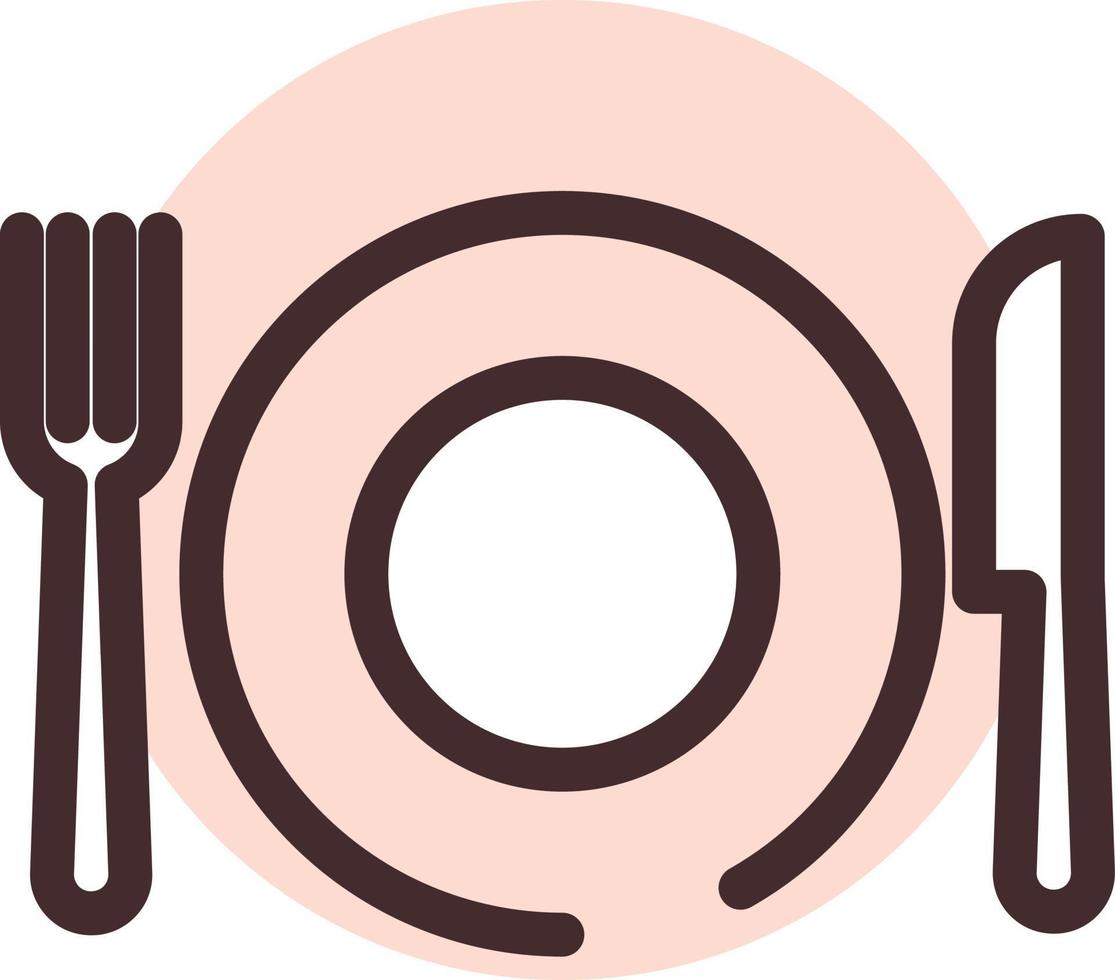The image is a graphic illustration commonly used as an icon on digital devices, depicting a dining setting. The central element is a large pink plate with two concentric circles, the outer one being slightly broken at the bottom right. The inner circle is white while the outer circle is a light orangish-pink hue extending into the fork and knife beside it. Positioned on the left is a white fork outlined with thick brown trim, and a similarly styled white knife on the right. The entire composition is set against a plain white background, which emphasizes the vibrant colors and bold outlines of the elements.